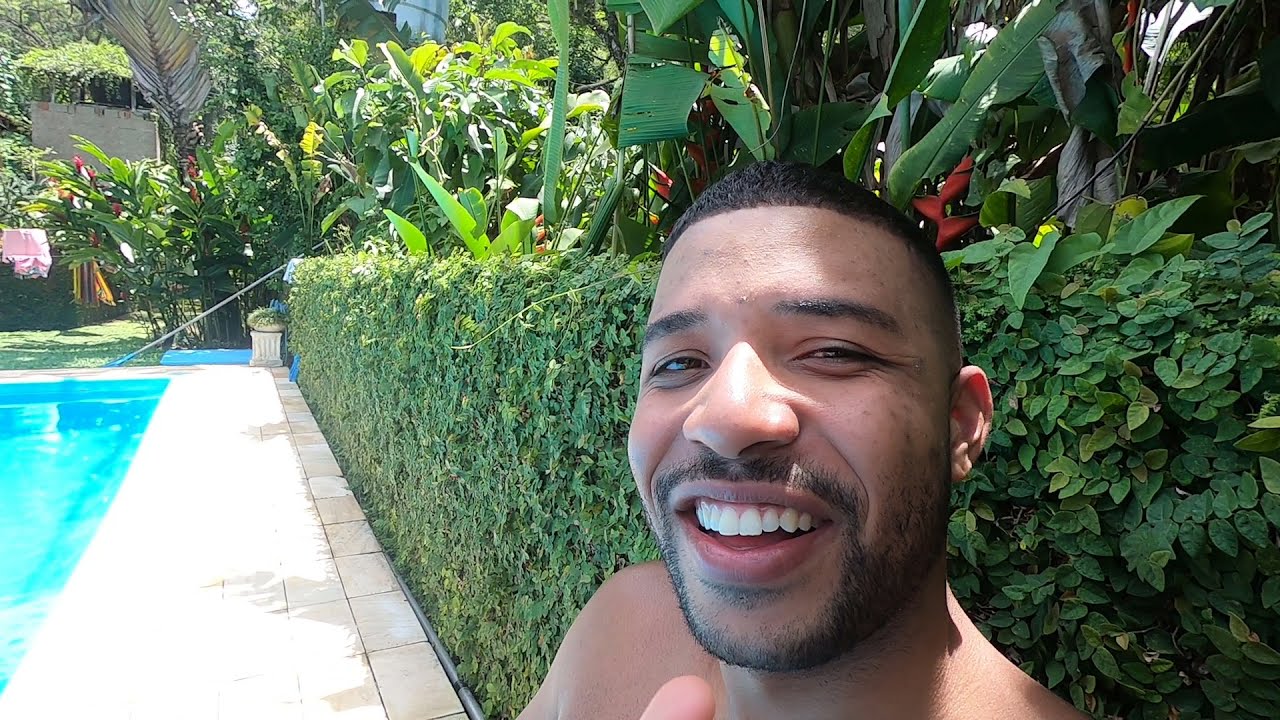In this image, we see a cheerful African American man taking a selfie outdoors by a clean, light blue in-ground pool. He has a beard, mustache, and short black hair, and he is smiling broadly, showing his teeth. He is sitting near a concrete sidewalk that encircles the pool. The background is lush with various well-manicured bushes, small plants, and trees with many green leaves and some flowers. Notably, there are canna-style plants and taller trees further in the distance. A concrete pot perched on a small pillar adds to the garden's charm. Visible beside the pool is a net for cleaning and a clothesline. A nearby building also makes an appearance in the background. The scene is captured during the daytime, possibly midday, with abundant sunlight illuminating the vibrant colors of green, blue, tan, and other hues in the garden.